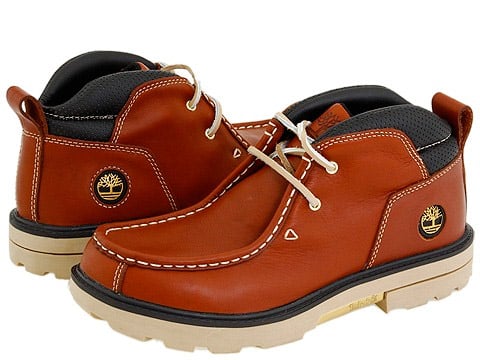The photograph depicts a pair of stylish, brown leather boots arranged in opposite directions on a solid white background. Both boots feature two rows of beige, rawhide-type shoe strings and sturdy cream-colored soles with black trim edges. Each boot is adorned with a circular, gold and black tree logo near the heel, likely indicating they are Timberland brand. Notable details include white stitching around the boots and a helpful loop on the back for easy wear. The heels are robust and beige in color, aligning with the overall rugged aesthetic while adding strong structural support. The interior of the boots is black, and they fit ankle-high, offering a versatile look that borders on hiking or casual use. No additional identifying information such as price or name is visible in the cropped image, emphasizing the boots themselves.